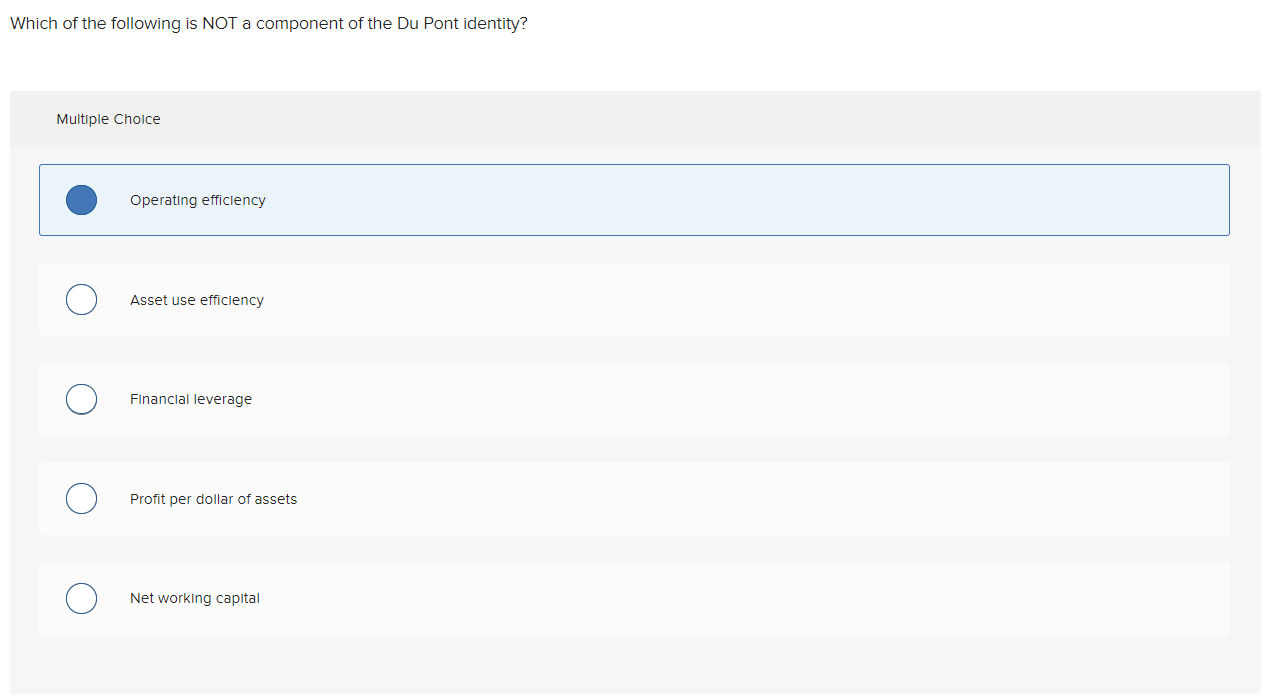The image presents a pale, simplistic design featuring seven short lines of text against an almost white background. The text is in a small, gray font, making it less prominent than typical black-on-white prints. At the top, the prompt reads: "Which of the following is not a component of the DuPont identity?" It's a multiple-choice question with five options listed below:

1. Operating efficiency
2. Asset use efficiency
3. Financial leverage
4. Profit per dollar of assets
5. Networking capital

The instruction is to identify which option is not a component of the DuPont identity. The selected answer in the image is "operating efficiency." The choice suggests that the other terms—asset use efficiency, financial leverage, profit per dollar of assets, and networking capital—are more integral parts of the DuPont identity.